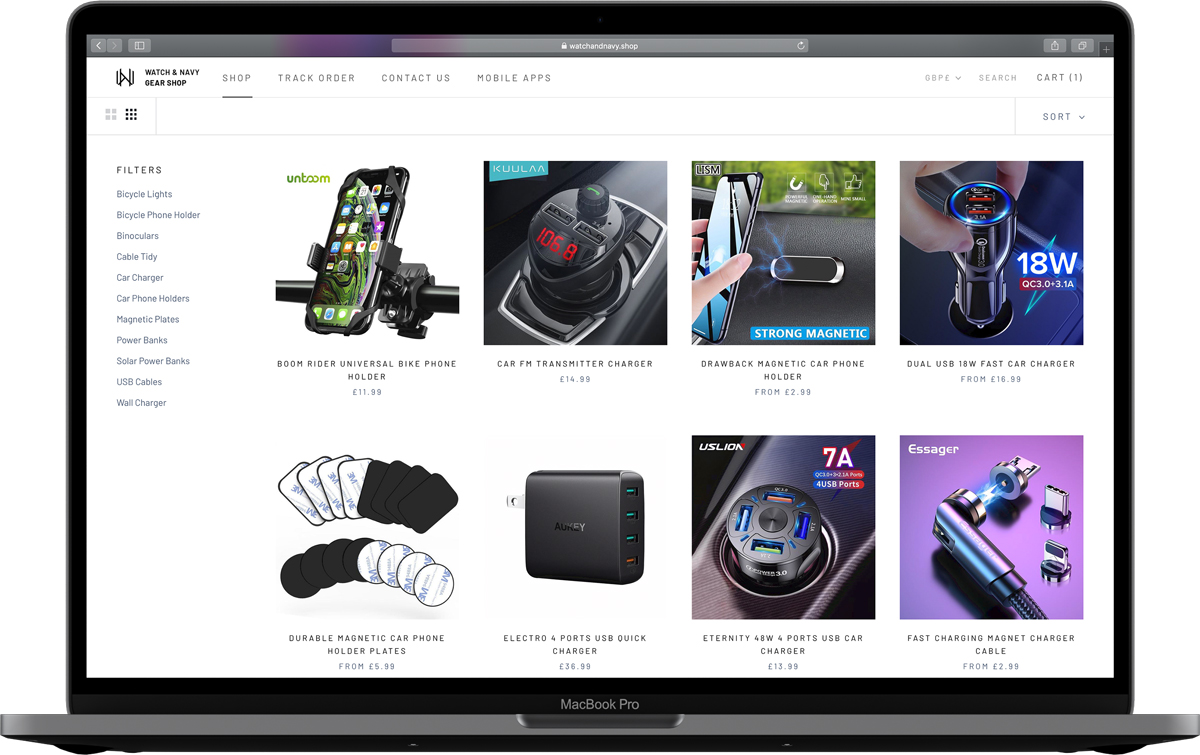Here is the cleaned-up and detailed caption:

"Displayed in the image is a MacBook Pro. The screen showcases a webpage from what seems to be an online tech store. Toward the top, on the left side, there are categories labeled as 'Watch,' 'Navy Dot Shop,' 'Navy Gear Shop,' 'Shop,' 'Track Order,' and 'Contactless Mobile Apps.' Below this is a series of filters and product listings.

On the left section of the screen, products such as bicycle eyes, bicycle phone holders, binoculars, cable tidies, various chargers, car phone holders, magnetic plates, power banks, solar prime banks, USB cables, and wall chargers are visible. 

Highlighted in the center is a promotion for a smartphone accessory, specifically a boomerang reverse back phone holder, priced at $11.99. 

The bottom section displays a variety of squares and circles depicting product icons, including a durable magnetic car phone holder starting at $5.99, a car transmitter charger at $14.99, a drawback magnetic car phone holder from $2.99, an 18W QC 3.0 charger, and dual USB 18W fast car chargers starting at $16.99. The section also lists an 'Electro 4.0 USB Quick Charger,' 'Eternity 4.0 USB Car Charger,' and a 'Fast Charging Magnetic Charger Cable' starting at $2.99.

In the bottom right corner, there is a visual element featuring a purple color."